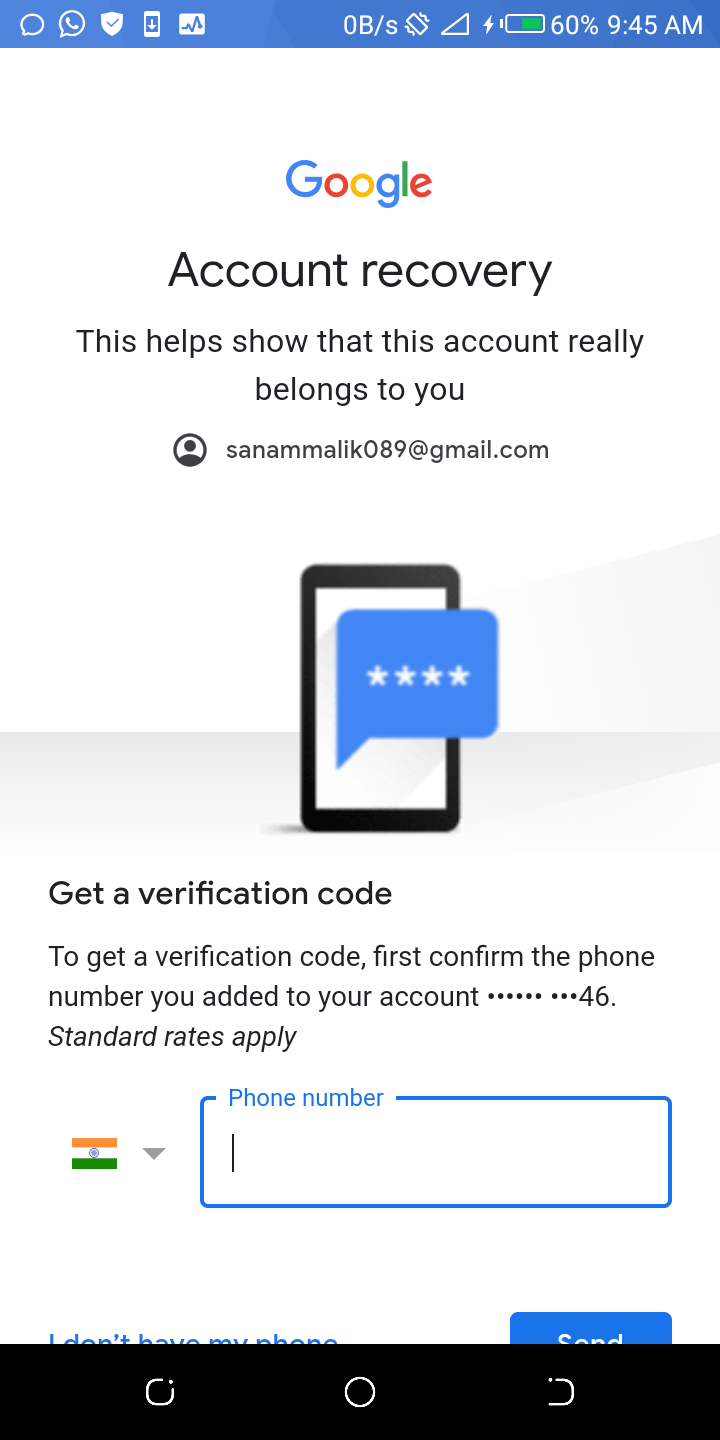The image appears to be a screenshot taken from a smartphone, featuring a blue border at the top. On the right side of the border, the battery icon displays 60 percent, and the time is shown as 9:45 AM. Below the border, the screen is predominantly white, with the Google logo and the title "Account Recovery" situated at the top.

Beneath the title, there is a message that reads, "This helps show that this account really belongs to you," followed by the email address "Sonomalik089@gmail.com." Further down, there is an image of a black box containing a blue conversation bubble with four stars in it.

The text continues to explain the process: "To get a verification code, first confirm the phone number you added to your account." Most of the phone number is obscured, except for the last two digits, "46," with a note indicating that standard rates apply.

On the left side of the image, there is a flag with horizontal stripes in yellow, white, and green. To the right of the flag, there is a text box for entering a phone number. Directly below this, there is a blue button labeled “Send.”